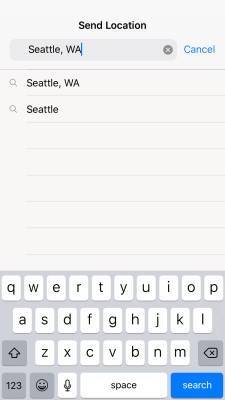This screenshot captures an iPhone displaying the interface for inputting and searching for a location. At the top of the screen, there are multiple elements: the "Send Location" button, a search field labeled "Search," and a text input box containing the phrase "Seattle, Washington." Adjacent to the text box are two buttons, "Cancel" and "Clear," which provide options to cancel the search or clear the inputted text, respectively. Below these elements, a list of search results is visible, featuring "Seattle, Washington" as the first result and simply "Seattle" as the second. Dominating the lower portion of the screen is the iPhone's keyboard, featuring a QWERTY layout. The keyboard includes keys for each letter of the alphabet, a shift key, a "123" key for numbers and special characters, an emoji key for emoticons, a microphone key for voice input, a space button, and a "Search" button to execute the search. The clean and intuitive design of the interface is characteristic of Apple's iOS, making it easy for users to quickly search and find locations.